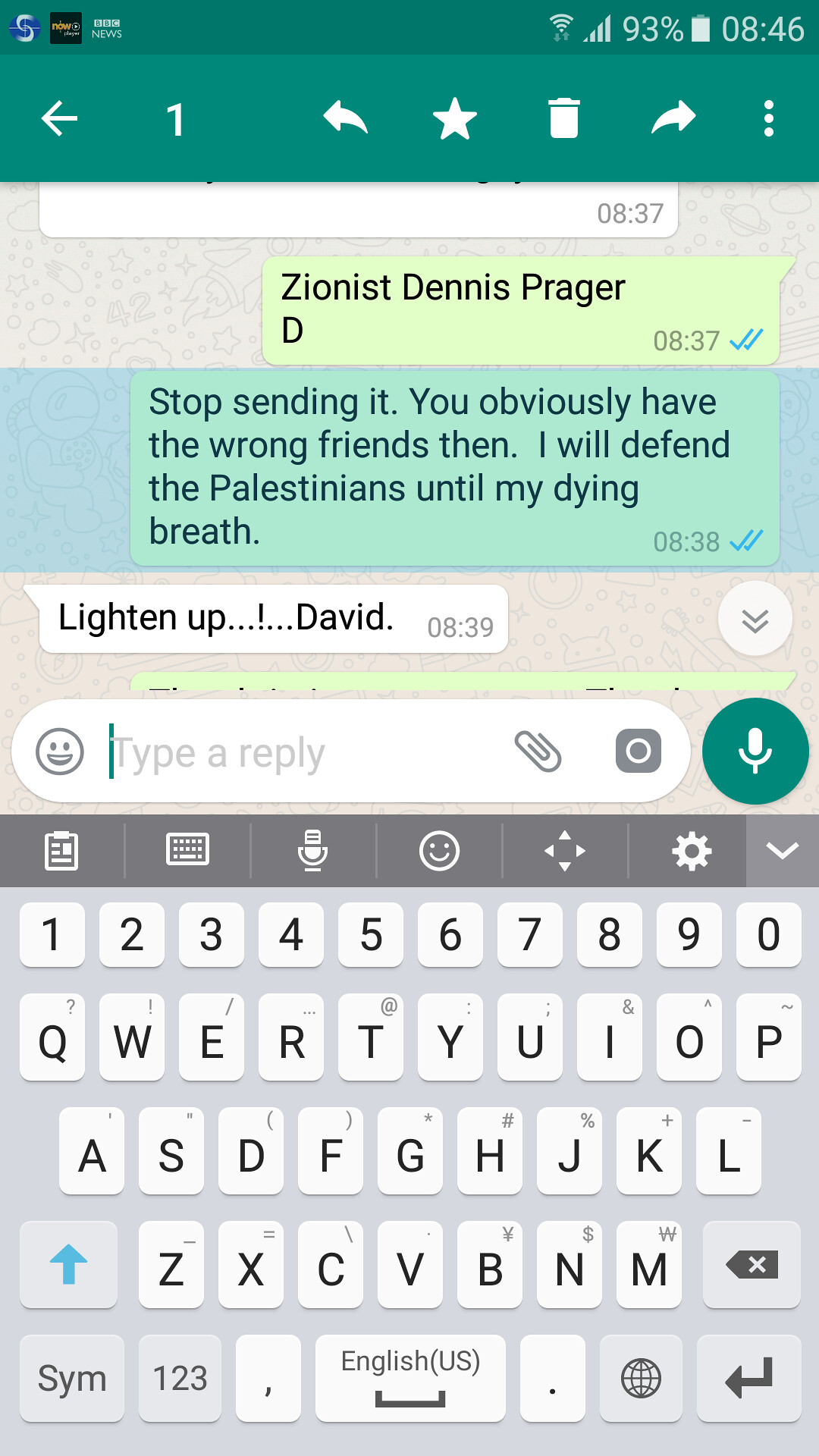This vertically aligned rectangular image is a screenshot captured from a mobile phone’s texting app. The dark green header at the top of the screen displays various icons including a left-pointing arrow, a number one, a thicker left-pointing arrow labeled "resend reply," a star, a trash can, a right-pointing arrow, and three vertical dots on the far right side. Below the header, the phone's status bar shows the Wi-Fi signal bars, a battery level of 93%, and the time, which is 8:46 AM.

The main section of the image features a conversation between two individuals. The first message, sent at 8:37 AM, in light yellow-green text reads, "Zionist Dennis Prager." This message is marked with two blue check marks, indicating it has been read. The subsequent message, sent at 8:38 AM, states, "Stop sending it. You obviously have the wrong friends then. I will defend the Palestinians until my dying breath." This message is also marked with two blue check marks. Following this, at 8:39 AM, another message in light yellow-green text simply reads, "Lighten up, David."

The bottom section of the screen shows a reply bubble that says "Type a reply," accompanied by a smiley face icon and a paperclip attachment symbol. Below that, the keyboard is visible, featuring numbers on the top row and letters on the bottom rows, all set against a gray background with each key lit up in a white square.